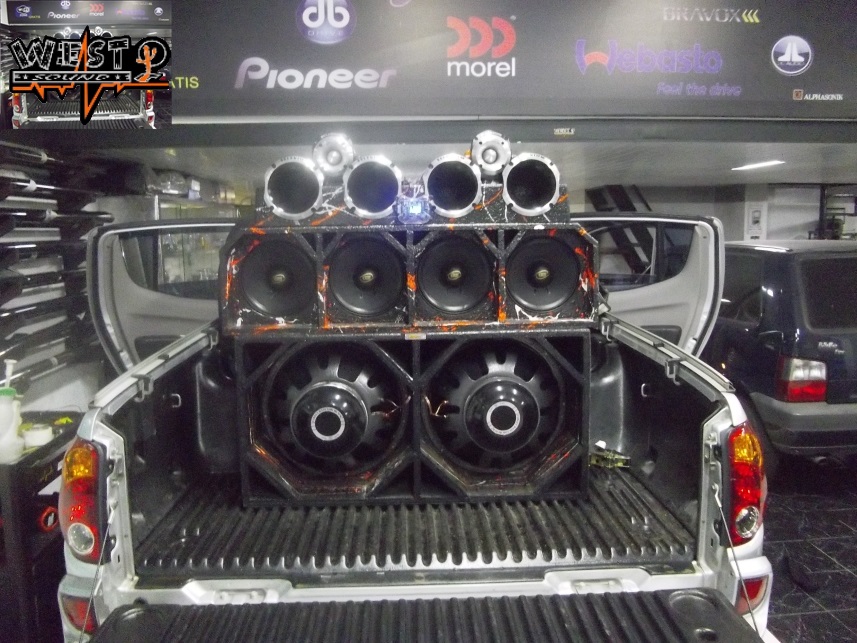This is a detailed color photograph of a car showroom, showcasing the custom audio setup in the flatbed of a white pickup truck. The image is taken from the back, with the tailgate lowered, revealing a black, ribbed liner designed to prevent objects from sliding. The truck's bed features an intricate arrangement of various speakers and tweeters mounted to the back of the front cab. Specifically, there are two large speakers with black rings and white centers at the bottom, four horizontally-aligned speakers with orange elements above them, and multiple silver-rimmed tweeters, some of which are positioned at the top of the setup.

To the left of the truck, a workbench with cleaning supplies on a small black tray is visible, and to the right, a dark blue SUV with a grey bumper is partially obscured. Above the truck, several logos from brands such as Pioneer, Morel, Webasto, and others are displayed, indicating the showroom's emphasis on vehicle customizations and accessories. The Pioneer logo appears in white text, the Morel logo includes red 'C's, and the Webasto logo features a distinctive 'W' with a red line through it followed by the text "Feel the Drive" in purple. This setting and arrangement suggest the showroom is advertising its ability to install advanced audio systems and other custom modifications for vehicles.